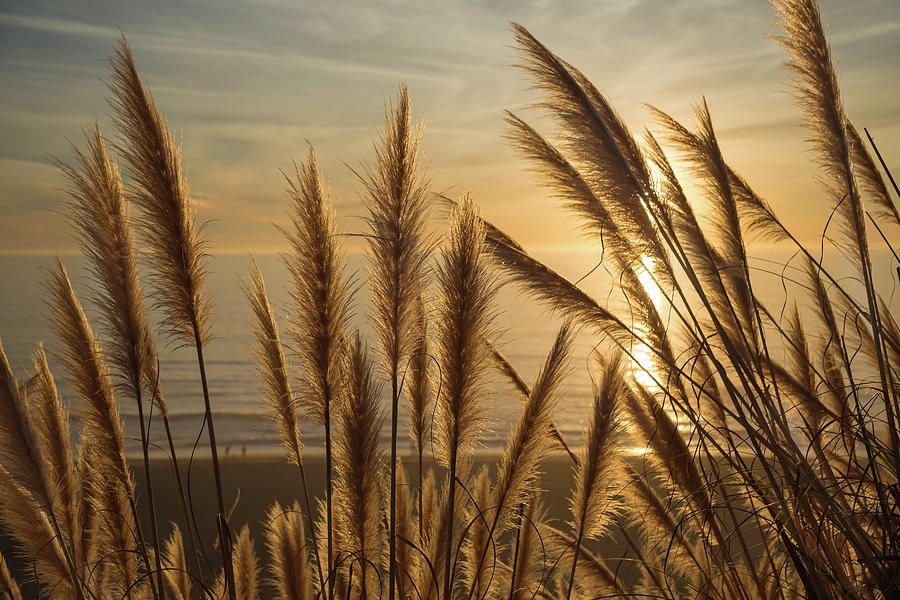This photograph captures a serene beachfront scene through a dense foreground of golden brown stalks, likely wheat or seagrass, gently swaying in the breeze. Between two of the stalks in the bottom-left corner, two people stand at the water's edge, adding a human element to the tranquil setting. The water is calm, gently lapping against the shore and reflecting the muted glow of the sun, which is partially hidden behind the stalks on the right. The sky, adorned with wispy cirrus clouds, is either bathed in the soft light of early morning or late evening, casting a yellowish hue across the horizon and the water. The overall atmosphere is peaceful and beautifully lit, with the sun's backlighting enhancing the natural colors of the scene.